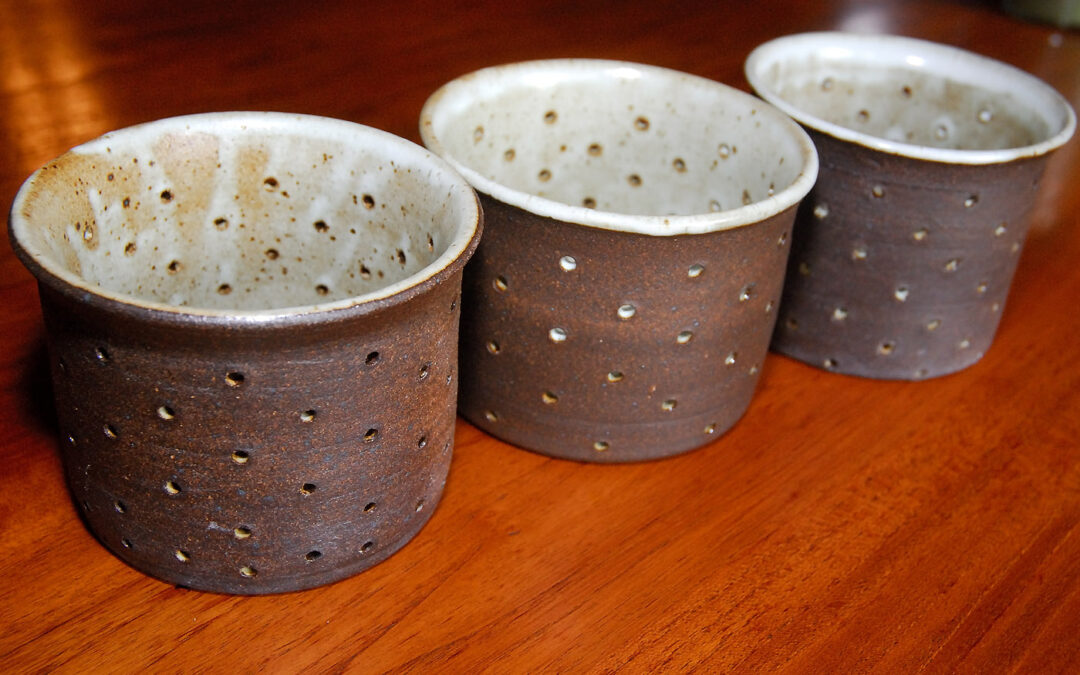The image features a close-up of three small, cylindrical containers made from what appears to be ceramic, arranged on a reddish wooden table. Each container has a rustic brown exterior and a white interior, with multiple small drainage holes around their sides, indicating they are likely used as plant pots. The interiors remain slightly stained, possibly from soil or coffee residue, adding to their worn, rustic appearance. The pots are touching each other, forming a slight diagonal line from the bottom left to the top right of the image. The consistently earthy tones and the positioning of the containers create a visually pleasing arrangement on the wooden surface.